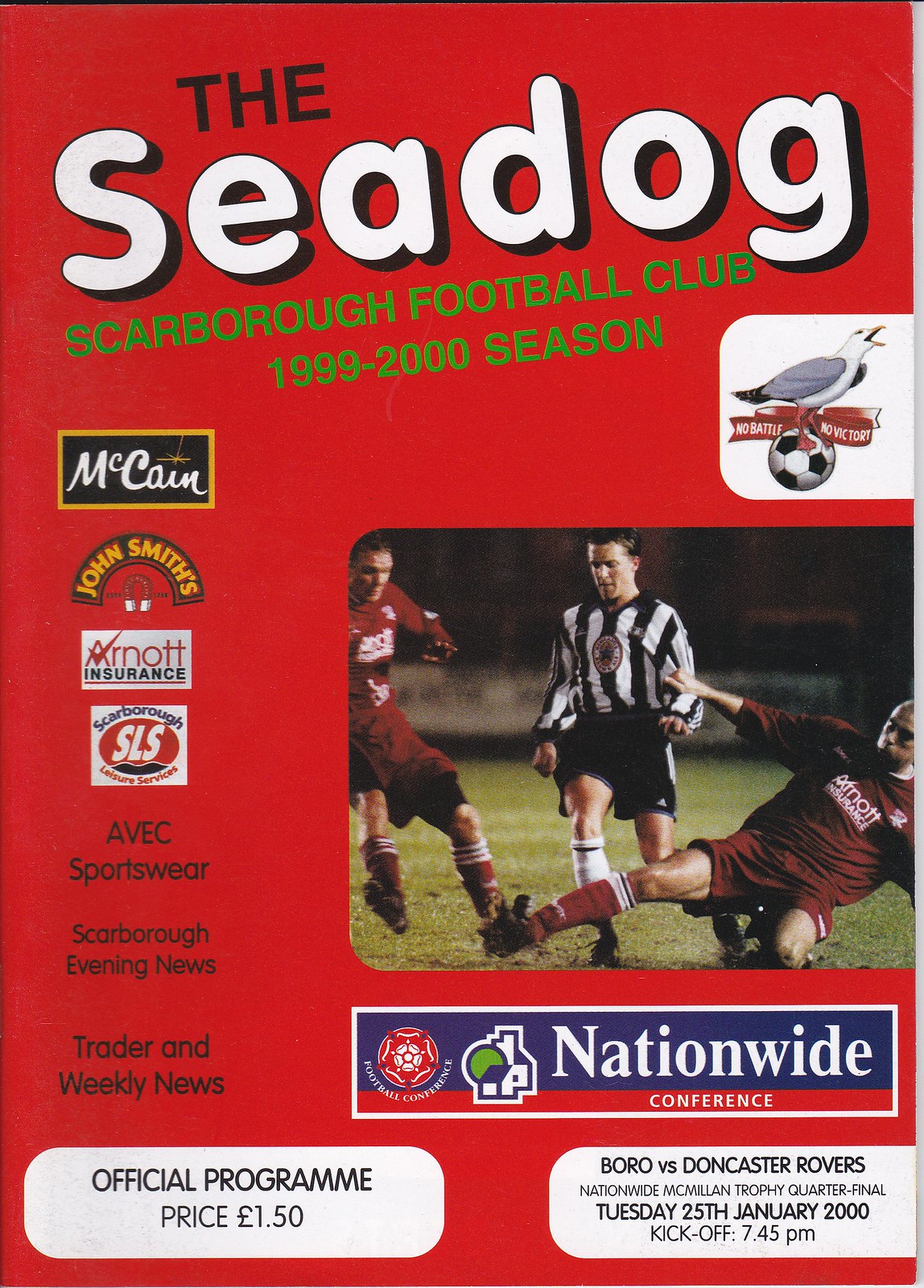The image depicts the cover of an official program for a Scarborough Football Club event during the 1999-2000 season. The entire background is red, with "THE SEADOG" prominently displayed at the top in large white letters with a black shadow. Beneath this, green text reads "SCARBOROUGH FOOTBALL CLUB 1999-2000 SEASON." 

On the right side of the cover, there's a detailed illustration of a white bird, possibly a seagull, with orange feet, a yellow beak, blue wings, and black wing tips standing on a black-and-white soccer ball. Further down on the right, a picture captures a moment from a soccer game with two players in red uniforms and a referee in black shorts and a black-and-white striped shirt. The game is set on green grass with a white wall in the background. Below the image, the text "NATIONWIDE CONFERENCE" is displayed, featuring symbols of a house and a tree in white, blue, and green.

On the left side of the cover, sponsor logos are arranged vertically: "MCCAIN" in white on a black and gold background, "JOHN SMITHS" in gold on black, "R-NOT INSURANCE" with "R-NOT" in red and "INSURANCE" in black on white, "SCARBOROUGH" in blue, "SLS" in white on red, "A-B-E-C SPORTSWEAR", "SCARBOROUGH EVENING NEWS," "TRADER," and "WEEKLY NEWS" all in black.

At the bottom left, the text "OFFICIAL PROGRAM PRICE £1.50" is written in black on a white background. On the bottom right, it announces the event details: "BOROUGH v. DONCASTER ROVERS NATIONAL MACMILLAN TROPHY QUARTER FINAL TUESDAY 25TH JANUARY 2000 KICKOFF 7.45 PM" in black letters on a white background.